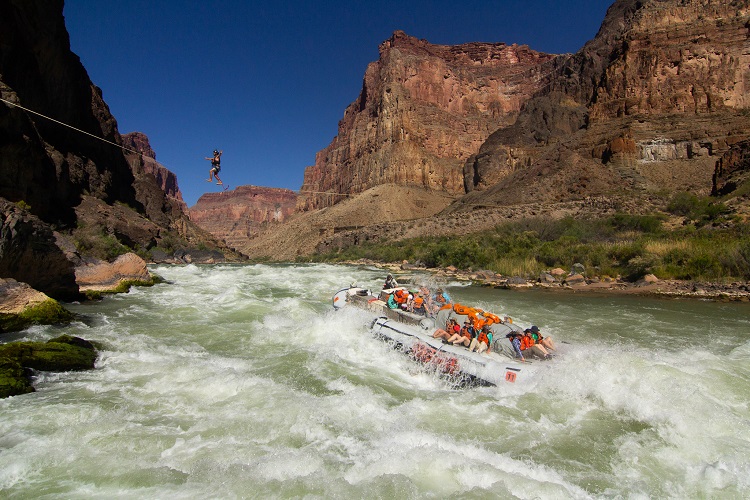In this captivating daytime outdoor photograph, the dynamic scene captured centers around a tumultuous river coursing through rugged, mountainous terrain, with mossy and rocky riverbanks. The river is flanked by towering rock formations and scattered greenery. At the heart of the image, a large, white raft braves the churning whitewater rapids, loaded with people clad in bright orange life jackets, their expressions a mix of excitement and trepidation as they're jostled by the restless waves. Above this thrilling aquatic adventure, a secondary yet strikingly daring spectacle unfolds: a woman meticulously traverses a tightrope stretched across the river, her arms extended for balance as she makes her way three-fourths of the distance to the opposite side. The clear blue sky provides a serene backdrop to this action-packed scene, accentuating the juxtaposition of natural beauty and human bravery.